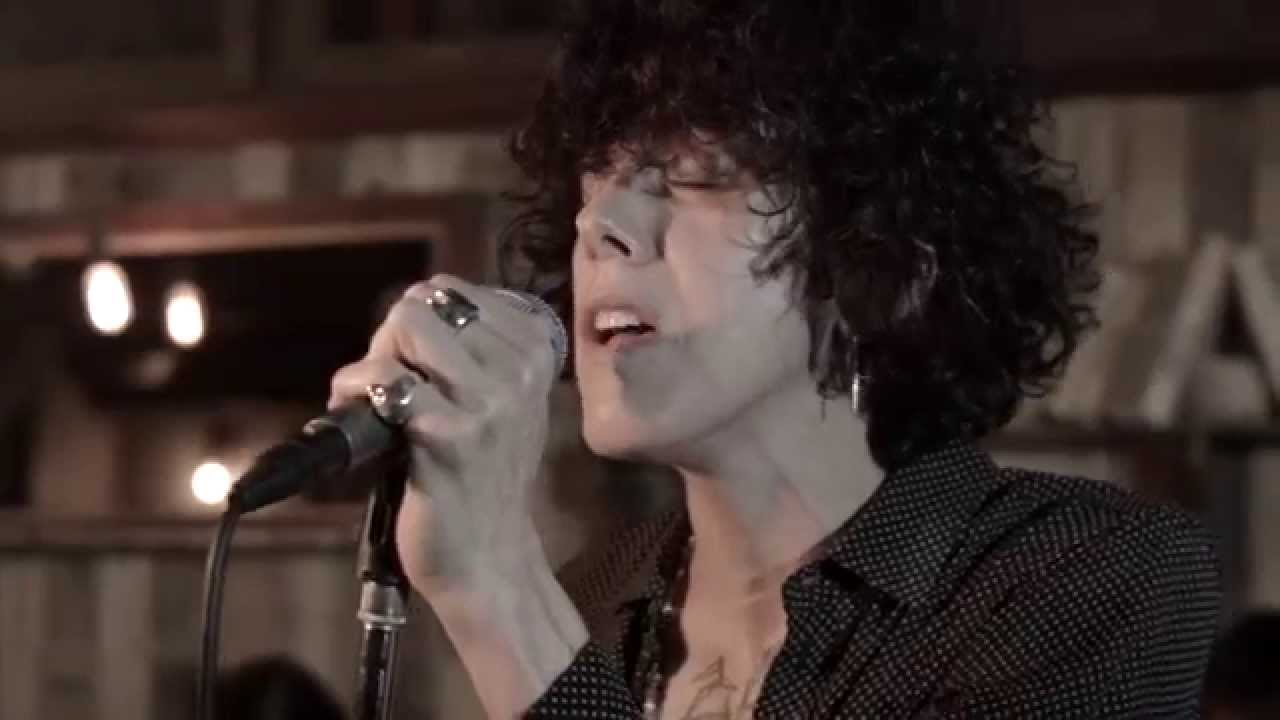The photograph captures a young male singer with medium-length curly hair, passionately singing into a corded microphone held in his left hand while his eyes are closed. He is adorned with a silver earring in his left ear, a necklace, and two rings—one on his pinky and one on his middle finger. He is dressed in a black, collared button-up shirt with white polka dots, which is unbuttoned at the top to reveal visible chest tattoos. The background is a slightly blurred studio setting with wooden walls and a large mirror reflecting sepia-toned lights, creating an intimate, soulful atmosphere.